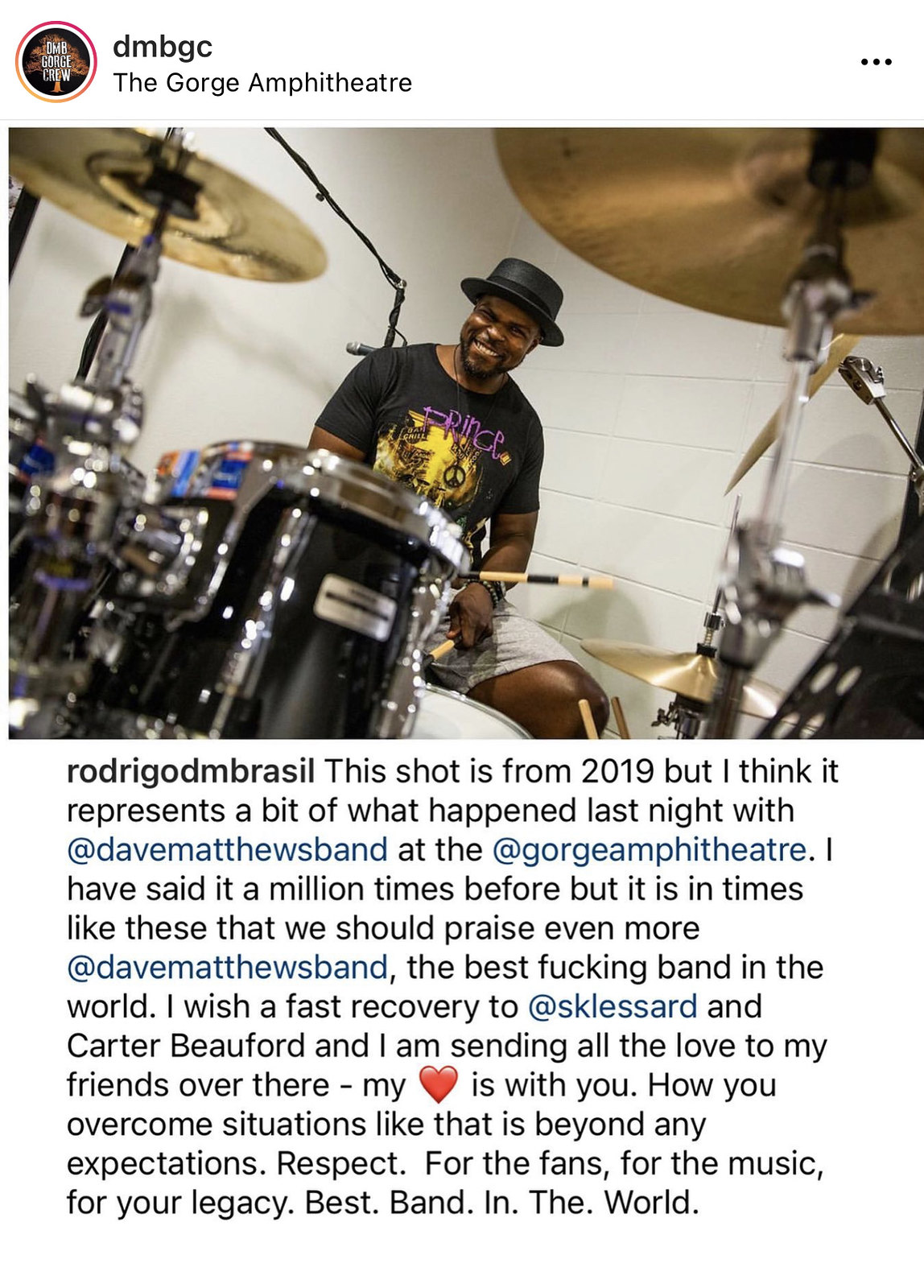The image showcases the Instagram post from DMBGC at the George Amphitheater. At the top, the username and venue information are displayed. The centerpiece is a photo of a young black man, likely in his 30s, wearing a black bowler hat and a black t-shirt with a yellow and purple logo. He is sitting beside a drum set, holding drumsticks, and smiling warmly. The drum set in the foreground includes a snare drum and two cymbals positioned at opposite corners.

Below the image is a caption that includes the name "Rodrigo D.M. Bracel." It provides context to the image and reads: "This shot is from 2019, but I think it represents a bit of what happened last night with the Dave Matthews Band at the George Amphitheater. I’ve said it a million times before, but it is times like these that we should praise the Dave Matthews Band even more. The best fucking band in the world. I wish a fast recovery to Sclessard and Carter Beatford. I am sending all the love to my friends over there; my heart is with you. How you overcome situations like that is beyond any expectations. Respect for the fans, for the music, for the legacy. Best. Band. In. The. World."